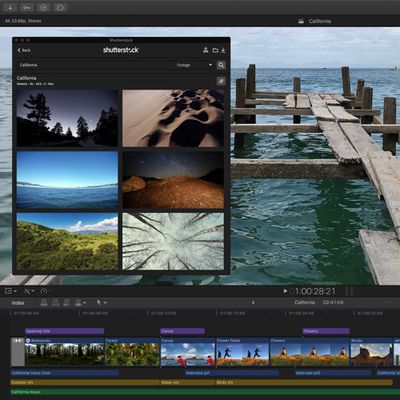The image depicts a screenshot of a video editing software interface in use. The timeline, located at the bottom, stretches to approximately one hour and 28 minutes, indicating the user is working on a relatively long project. The timeline is segmented into several sections, each marked by thumbnails representing different scenes or segments of the video. 

Due to the blurriness of the image, specific text is not legible, but the variety of colorful horizontal strips along the timeline likely denote different elements or features within the video, such as audio tracks, transitions, or effects. The extensive tool panel at the bottom displays a wide array of video editing tools, suggesting robust functionality.

Above the timeline, there are numerous template images, implying that the software offers customizable options for enhancing the video. Overall, the interface brims with options and detailed editing capabilities, providing the user with extensive control over their video project.